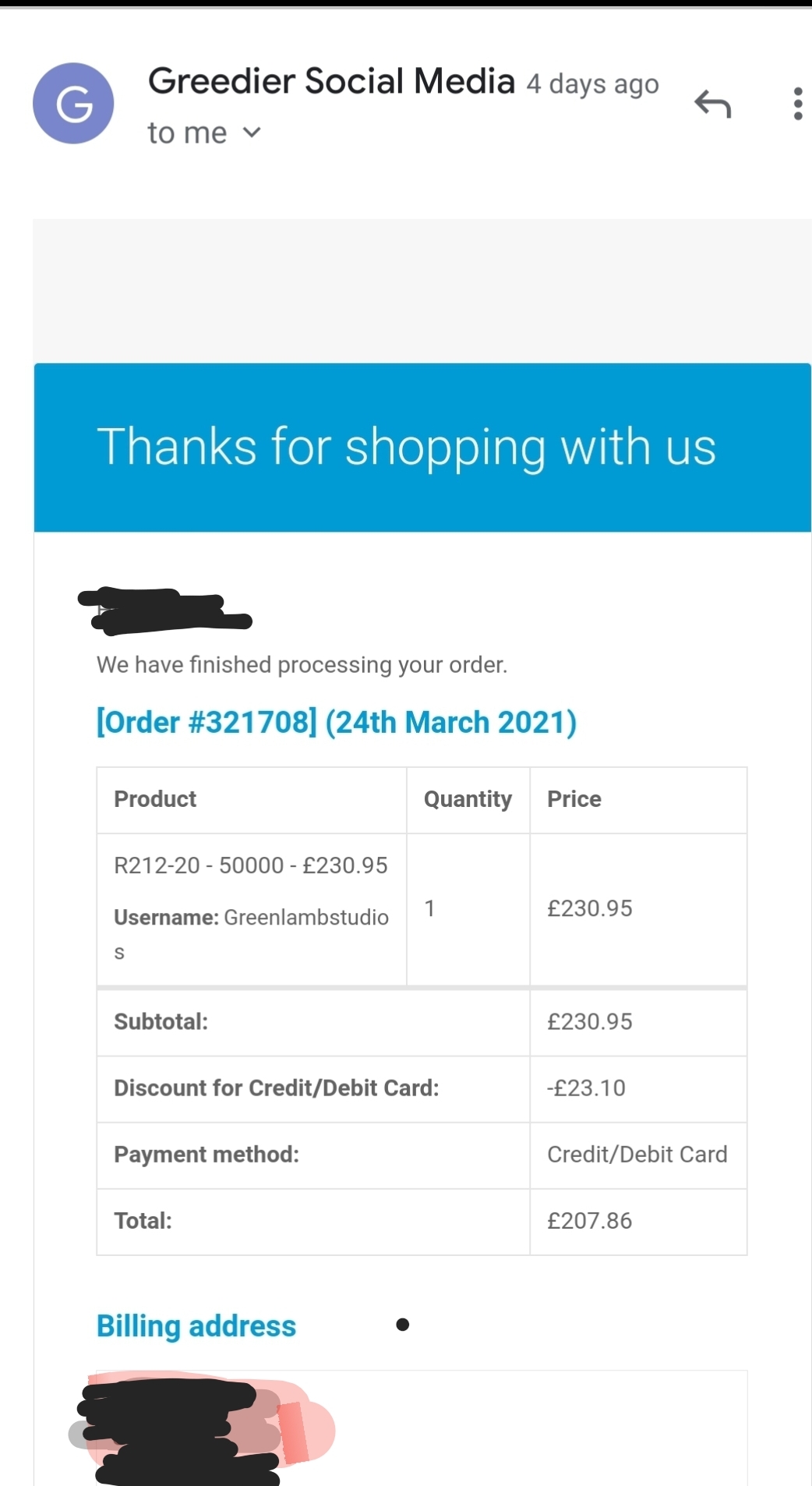The screen image displayed is a digital receipt for an online purchase from a specific website, prominently featuring elements of a social media overlay. At the top, it shows a notification from 'Greedier Social Media,' dated four days ago, next to a profile picture depicted as a simple purple circle with a white 'G' inside it. Below this, there is an interactive element labeled 'To me' with a drop-down arrow.

In the main body of the receipt, a prominent blue box with white writing extends thanks to the customer, stating "Thanks for shopping with us." Beneath this, some text is blacked out, followed by a confirmation message, "We have finished processing your order." The receipt details the order with number '321708,' processed on March 24, 2021.

The receipt itemizes the purchase, displaying the product as 'R2 1 2 2 0 5 0 0 0 0,' purchased in the quantity of one, at a unit price of £230.95. The username associated with the order is 'greenlamstudios.' The total cost of the product comes to £230.95, with a discount for using a credit/debit card amounting to £23.10. The payment method noted is via 'Credit/Debit.' After applying the discount, the final total is £207.86. The billing address section is entirely obscured with black, peach, and purple markers, ensuring the personal details are not visible.